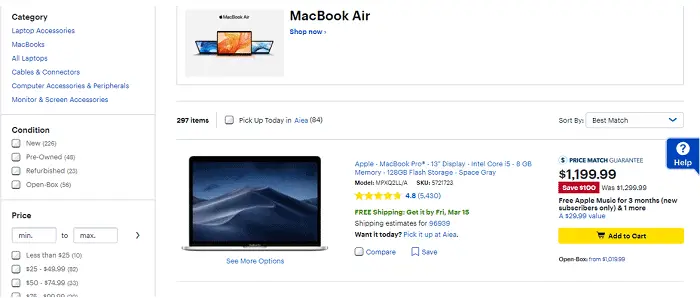A user navigates a retail website intending to purchase a MacBook Pro. They add to their cart an Apple MacBook Pro with a 13-inch display, powered by an Intel Core i5 processor, featuring 8 GB of memory and 128 GB of flash storage in the color Space Gray. The model number is NPX02LL/A, and the SKU is 5721723. This laptop has received 4.8 stars based on 5,430 reviews. The item qualifies for free shipping, with an estimated delivery date of Friday, March 15th, for the zip code 90539. There is also an option to pick up the laptop the same day at a store in Aiea, Hawaii, suggesting the retailer could be Best Buy. The laptop is priced at $1,199.99, reflecting a $100 discount from its original price of $1,299.99. Additionally, new subscribers can enjoy three months of Apple Music for free.